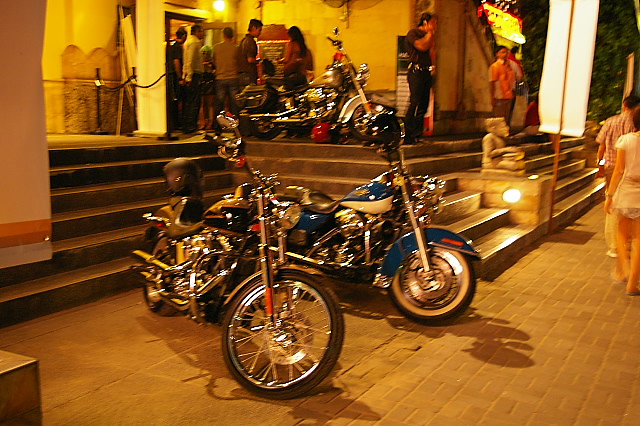This captivating photograph showcases three gleaming Harley-Davidson motorcycles parked in front of a sophisticated nightclub in Spain, exuding a distinct Spanish ambiance. The motorcycles, primarily blue and white, black, and white, have highly polished chromes and lustrous wheels, drawing the attention of passersby. In the foreground, a man dressed in dark attire is engaged in a phone conversation on the sidewalk. The scene is bustling with people, some casually strolling by, others entering or exiting the nightclub via a set of stairs leading to the entrance. Illuminated by the club's stylish lights, the overall setting emanates a tranquil yet lively atmosphere, capturing a moment of social interaction and urban elegance.